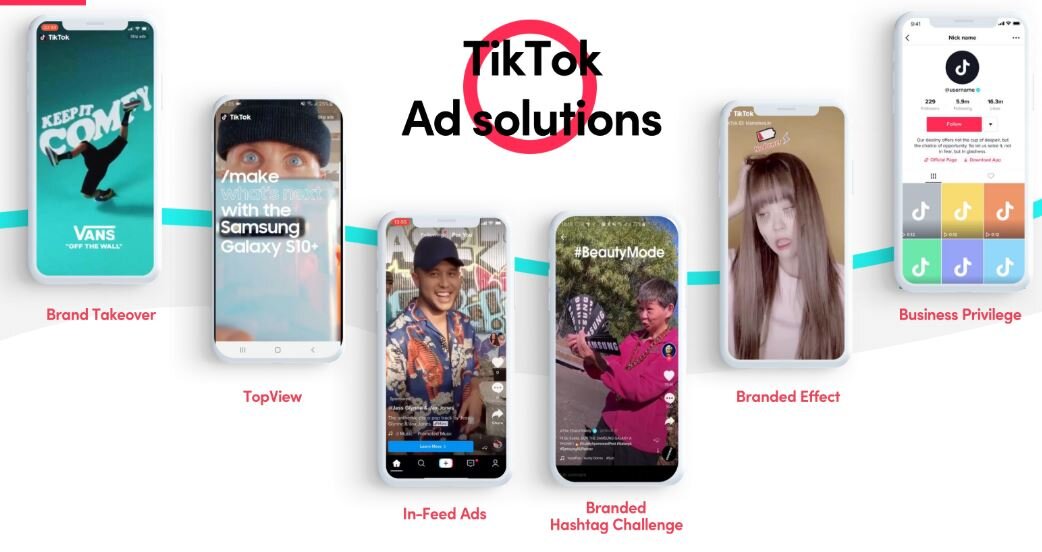This promotional graphic illustrates TikTok Ad Solutions, with a prominent red circular highlight around the text. The image details six distinct TikTok ad formats, each demonstrated by a smartphone screen displaying an example of the respective ad.

1. **Brand Takeover**: Features a person performing a dance accompanied by the text "Keep It Comfy" and the "Vans Off The Wall" branding.
2. **Top View**: Showcases a close-up of a person's face with the text, "Make What's Next With Samsung Galaxy S10+," promoting the Samsung Galaxy S10.
3. **In-Feed Ads**: Depicts a person engaging with the camera in a casual setting. This ad type appears within the user's feed, resembling organic content, and includes engagement options such as likes, comments, and shares.
4. **Branded Hashtag Challenge**: Displays a person holding a product accompanied by the hashtag #BeautyMode.
5. **Branded Effect**: Shows a girl with long hair using a branded filter that applies makeup effects to her video.
6. **Business Privilege**: Presents a TikTok account overview, featuring a user profile screen, showcasing follower counts, likes, and content thumbnails.

The graphic effectively highlights the variety of ad formats available on TikTok, emphasizing their seamless integration into the platform's user experience.